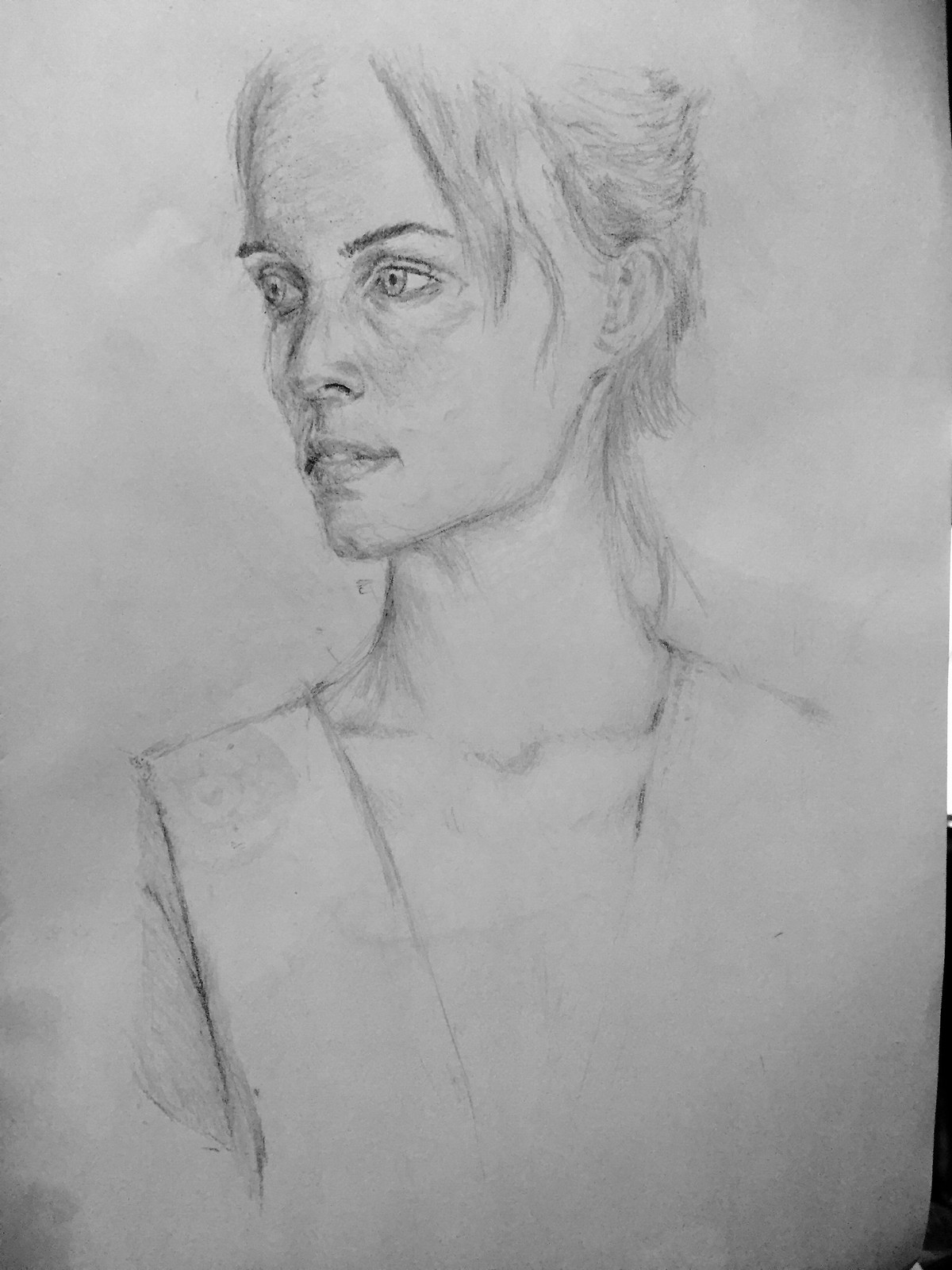The image is a detailed pencil drawing on plain white sketch paper, featuring a portrait of a woman with her head partially cropped out. She has short, blonde hair parted in the middle and styled to fall slightly over her eyes, with strands framing her face and pulled back. Her face, characterized by a slender jawline, is turned to the left side of the page with well-drawn features, including light-colored eyes, thin, well-manicured eyebrows, and a properly proportioned nose. Her slightly open lips reveal a hint of her teeth, contributing to an expression that seems slightly tired. Her neck and collarbones are distinctly shaded, extending down to a sleeveless shirt with a V-neck, revealing part of her upper chest. The drawing excels in detail around the eyes, nose, and mouth, adhering to the natural human focus on these features. This black-and-white portrait manages to capture both the structure and subtle expressions of the subject, reminiscent of Charlize Theron.